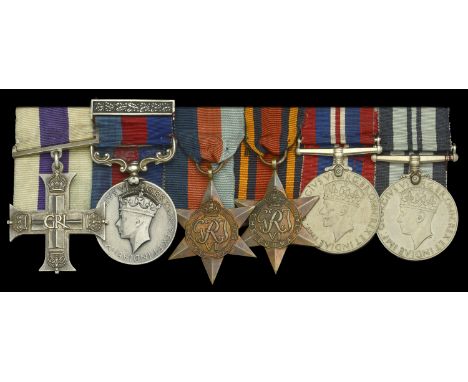The image depicts a collection of six distinguished military medals, each representing commendations likely from various countries. Starting from the left, the first medal features a silver cross, possibly an Iron Cross, suspended from a purple and white striped ribbon, with an inscription that appears to read "GRI." The second medal is circular, showcasing a side profile of a crowned man, likely a king, attached to a ribbon with blue, red, and blue stripes. The third and fourth medals are both six-pointed bronze stars, each prominently featuring a small central circle with the initial "R." The third medal's ribbon is decorated in blue, butterscotch, and white stripes while the fourth one is yellow, blue, and red. Completing the collection, the last two medals are circular medallions echoing the king's profile motif seen earlier. These medallions appear to be inscribed, possibly in Latin, and are mounted on ribbons—the fifth one with red, blue, and white stripes, and the final one on a gray and light blue striped ribbon. The medals' arrangement and varied ribbon patterns highlight their diverse and likely international origins.